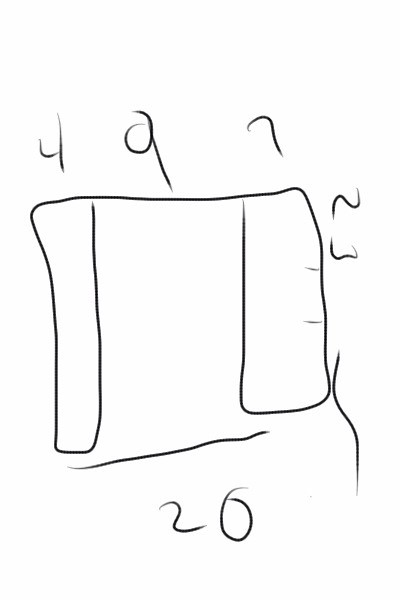This image appears to be a computer-generated drawing featuring various geometric shapes and numbers. At the top, there are a series of somewhat scribbled numbers: 4, 9, and 7, followed by a 23 positioned towards the right side. In the lower area of the image, the number 20 is prominently displayed in black. The drawing includes an uneven square situated near the center, accompanied by a rectangle to its side. Another rectangle shape lies to the right of this configuration. Additionally, a squiggly line is present to the far right. At the bottom, just above the number 20, a long, horizontal line extends across the image.